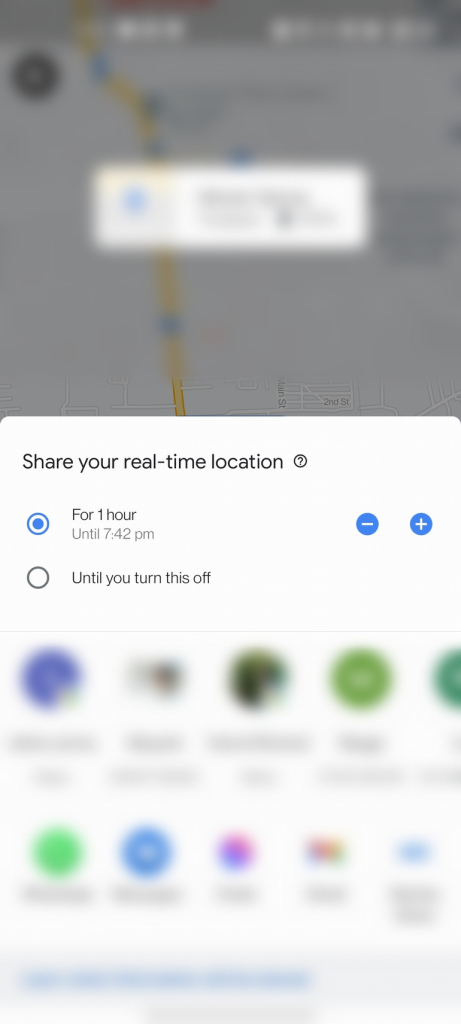The image displays a blurred map interface with a prompt titled "Share Your Real-Time Location." At the top of the interface, there is a black bar containing illegible white text. Below this bar, the majority of the map is obscured, save for a vertical road running north to south. 

Central to the image, a white overlay box serves as the main interactive area. The prominent text "Share Your Real-Time Location" is displayed, accompanied by a small question mark icon suggesting additional information upon interaction.

Beneath this, two buttons offer time options for sharing the location. The first button, highlighted in blue, is labeled "For 1 hour." Directly below it, the text reads "Until 2:42 PM," indicating the exact time the sharing will conclude. The second button is labeled "Until you turn this off," providing an indefinite sharing option. To the right of these buttons, blue plus and minus signs allow for time adjustments.

Further down, the interface appears to list contacts, though the names are blurred and difficult to read. One contact is highlighted in blue, suggesting it is selected. The rest appear as standard text, possibly referencing additional contacts from the user’s phone.

At the very bottom of the interface, additional text in blue hints at a hyperlink, though its content is unreadable due to the blurriness. The only clearly visible text is the "Share Your Real-Time Location" directive, emphasizing the main function of the screen.